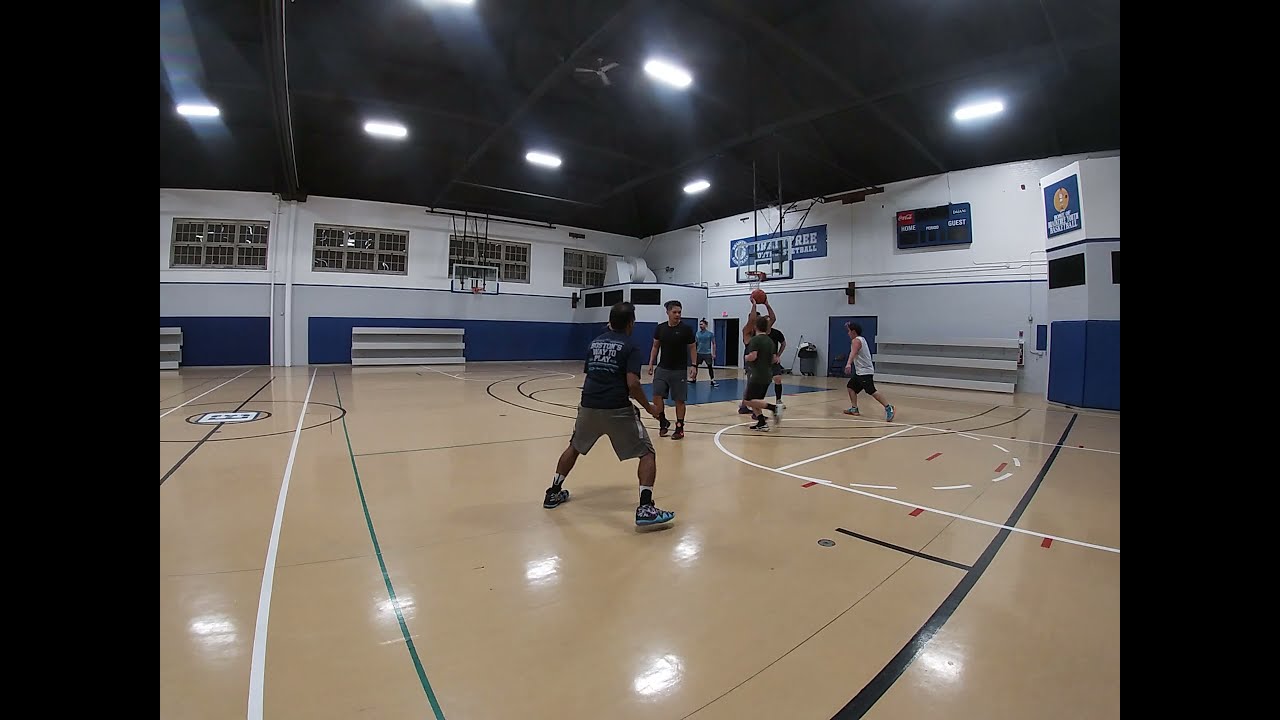The image captures an indoor basketball game taking place in what appears to be a high school gymnasium. Seven players are on the court, engaged in an informal practice session without uniforms. The gym features distinct walls—navy blue at the bottom, with light gray above. The upper sections of the walls have white sections with three small rectangular windows grouped in two rows, framed in brown. A man in a light blue shirt and black pants stands in the far background. In the foreground, a player in dark gray shorts and a navy blue shirt is visible. Another player, facing away from the camera, wears a blue shirt and tan pants, while his teammate in a blue shirt and khaki shorts faces the camera. Nearby, a player in a white t-shirt and black shorts is seen running. One player lifts the basketball high above his head, ready to make a play. The ceiling is dark with white lights illuminating the court. On the back wall, a banner with white writing and an unlit blue scoreboard are visible, alongside some illegible writing. The floor showcases the standard markings of a basketball court, enhancing the competitive atmosphere of the scene.